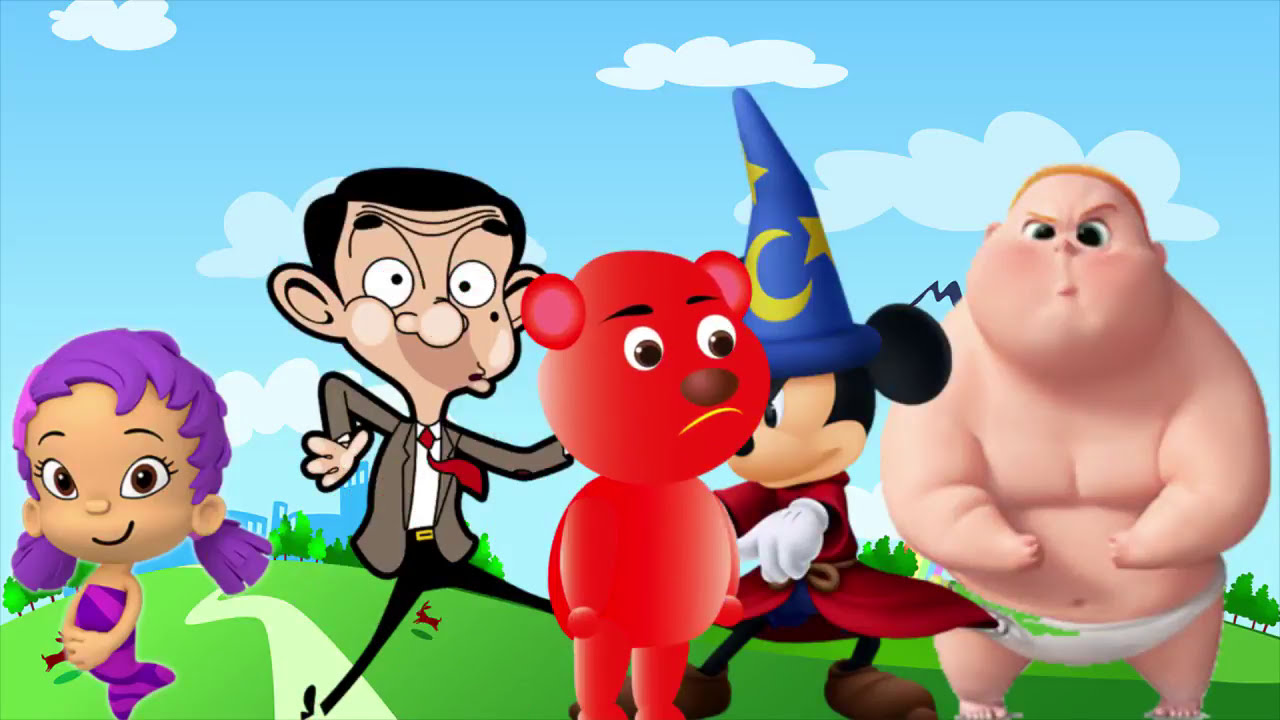In this vivid cartoon scene, a collection of iconic characters, each drawn in distinctive styles, stands together on a lush, grassy field under a clear, sunny sky with puffy white clouds. To the left, a small mermaid girl with tan skin and brown eyes displays a gentle smile. She features vibrant purple striped mer-tail that reaches just under her arms and her pink and purple pigtails add a touch of whimsy. Her hands are delicately folded in front of her. Adjacent to her is a cartoon version of Mr. Bean, distinguished by his exaggerated features, including a bulbous nose, big round eyes, and a comically bewildered expression. He wears a gray jacket, black pants, a red tie, and a white shirt. His thin legs and awkward posture contribute to his humorous demeanor.

In the center stands a red bear-like creature with a round body and head. The bear's expression is notably sad or concerned, indicated by its yellow frown and brown nose. Positioned slightly behind the bear is a three-dimensionally rendered Mickey Mouse, dressed as a wizard. Mickey is adorned in his iconic red wizard robe, brown shoes, white gloves, and a blue wizard hat embellished with yellow crescent moons and stars. His expression is serious, matching his grandiose attire.

To the far right of the group is a large, muscular baby, clad only in a white diaper. His face, with its large, asymmetrical eyes and raised left eyebrow, portrays a mix of confusion and anger. The baby’s short blonde hair, pronounced chin, and robust build add to his intimidating yet comedic appearance. This ensemble image captures a whimsical outdoor gathering of beloved characters, each distinct yet harmoniously composed within the bright, cartoonish landscape.